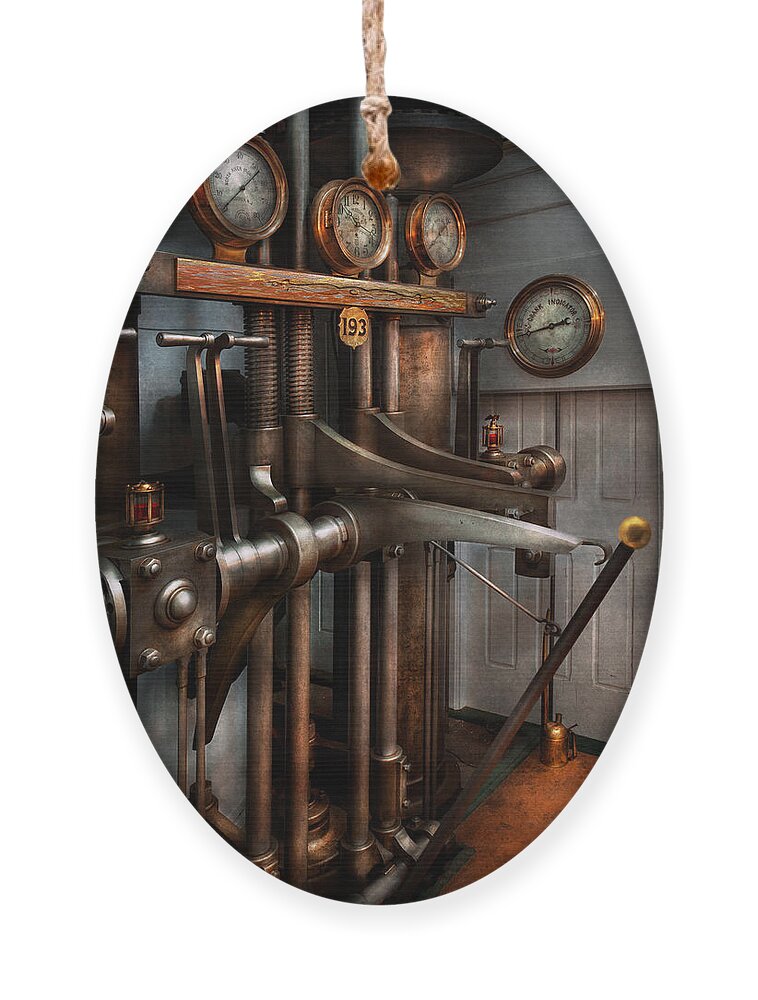The image is an intricately detailed, generated photo of an engine control room, framed in an oval shape and potentially resembling a Christmas ornament hanging by a string. The room is filled with mechanical components, including three to four gauges positioned at various points like the top right, bottom left, and around the nine o'clock mark. There are several levers—five to six in total—some of which suggest the machine is powered on. The scene includes an oil can on the floor and features some rusting parts, indicating wear and use. The backdrop consists of white wooden walls or a door, contributing to an industrial aesthetic. The number "193" is notably visible, adding a sense of specificity to the machinery. Overall, it depicts a highly detailed and operational industrial mechanism, though its exact function remains uncertain.